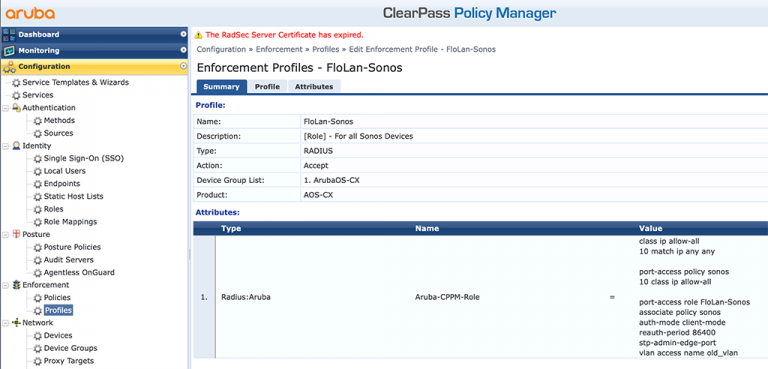Screenshot of a Desktop Application Interface Displaying Aruba ClearPass Policy Manager

The image captures a screenshot of the Aruba ClearPass Policy Manager application on a desktop. The interface showcases several key components and features of the software.

On the top-left corner, there is an indication that this is the Aruba OS. At the top-center, the title reads "ClearPass Policy Manager," confirming the specific software in use. 

The left sidebar functions as a navigation menu and includes several sections:

- **Dashboard**
- **Monitoring**
- **Configuration** (This section is expanded to reveal its sub-menu items):
  - Service Templates and Wizards
  - Services
  - Authentication
  - Methods and Sources
  - Identity (Expanded to show):
    - Single Sign-On
    - Local Users
    - Endpoints
    - Static Host List
    - Roles
    - Role Mappings
    - Posture
  - Posture Policies
  - Audit
  - Service
  - Servers
  - Agent List
  - OnGuard
- **Enforcement** (Currently highlighted and expanded to show):
  - Policies and Profiles
- **Network**
  - Devices
  - Device Groups
  - Proxy Targets

The main window on the right is focused on "Enforcement Profiles" and includes detailed information with columns labeled:

- Name
- Description
- Type
- Action
- Device Group List
- Product

This detailed view offers a comprehensive look into the enforcement profiles, showcasing how the ClearPass Policy Manager organizes and displays policy enforcement details within its application interface.